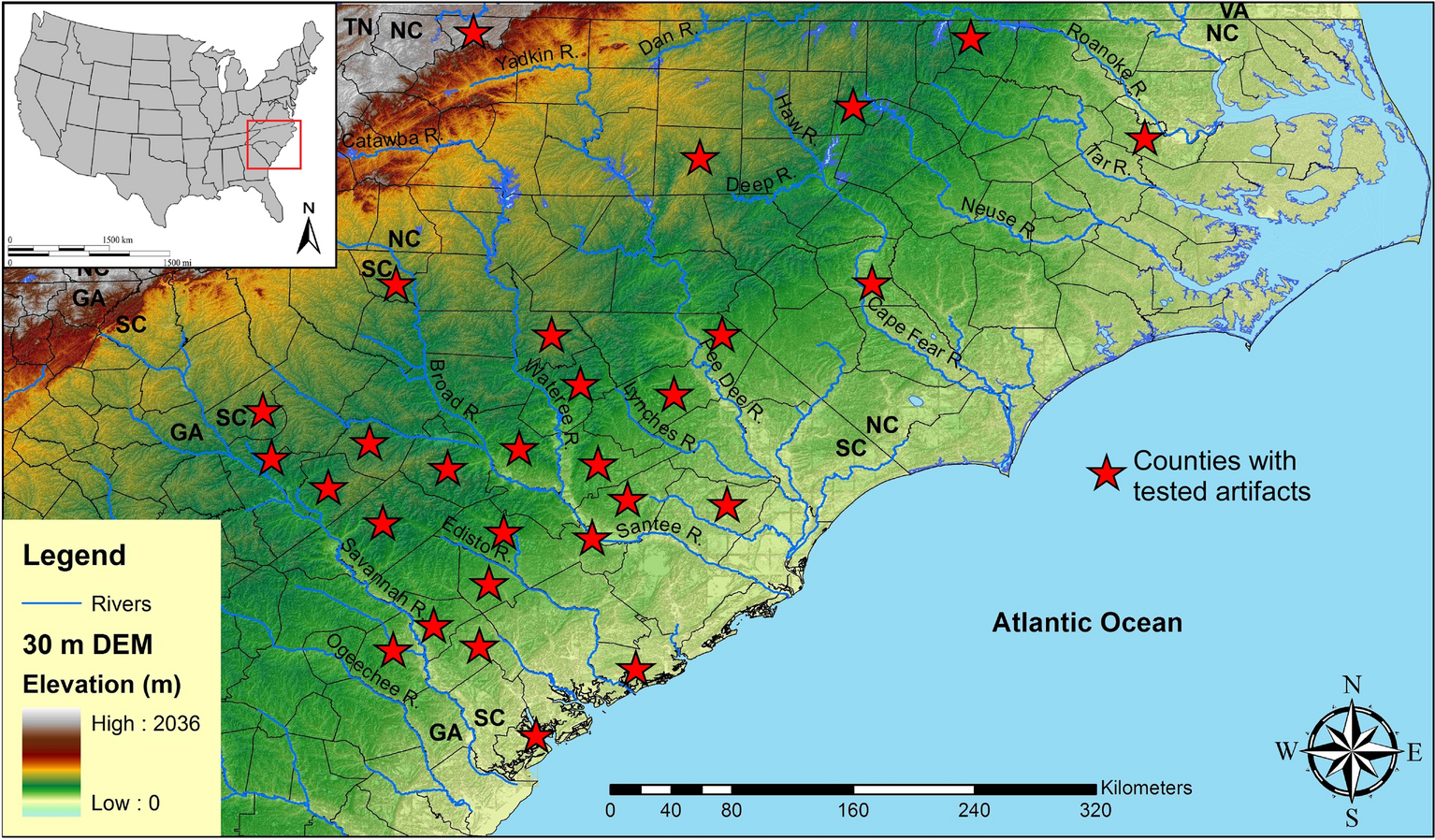This detailed photograph showcases an inset from a larger map, zooming in on the geographic region encompassing the lower part of Virginia, North Carolina, South Carolina, and the upper portion of Georgia. The map is notable for its topographical details and color distinctions to denote various elevations, from the pale green of the coastal plains to the dark browns of the mountainous areas. Red stars are scattered throughout the map, indicating counties with tested artifacts, as explained in the legend located in the lower left corner. Also, on this legend are depictions of rivers marked with gray lines and further defined by different colors representing elevation levels, with specific mentions of 30-meter DEM (Digital Elevation Model) data.

In the upper left corner, a smaller inset map with a white background highlights the entire United States in gray, with black outlines separating each state and a red square pinpointing the enlarged area of focus. The lower right corner of the map, overlaid on the blue Atlantic Ocean, features a black and white compass rose indicating the cardinal directions of North, South, East, and West (NSEW). The map also outlines counties and includes various rivers and lakes, accurately showing the physical and geological landscape of the specified region in vivid color. The use of elevation colors ranges from blue, representing the lowest levels, to a reddish-white depicting the highest elevations, creating a comprehensive and educational depiction of the area.